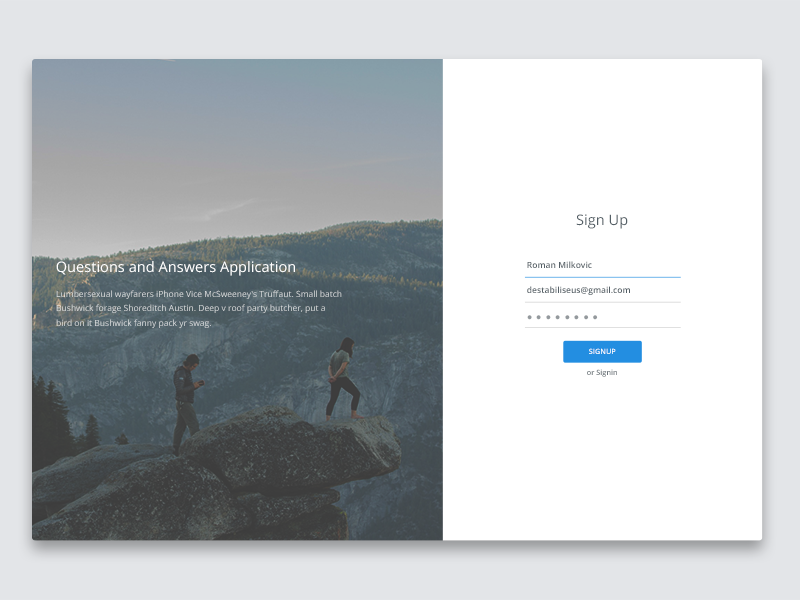This landscape-oriented photo captures a sign-up page for an app or website, set against a grey background that is slightly wider than it is tall. Central to the image is another rectangle, also landscape-oriented and divided into two sections. The larger section, occupying about two-thirds of the rectangle, features a vibrant sunset over a mountain range, with silhouetted figures standing on the edge of a rocky cliff. Among these figures is a person with shoulder-length hair on the right and another individual looking downward to the left. Centered in this colorful backdrop, white text reads "Question and Answers Application," with a smaller line of text below stating "Lumbersexual Wayfarer's iPhone."

On the right third of the rectangle, set against a white background, is the black text detailing the sign-up process. The username "Roman Milkovich" is displayed, followed by fields for an email address and a password, with the password shown as redacted dots for privacy. Below these fields, a blue rectangular button with yellow text invites the user to "Sign-Up."